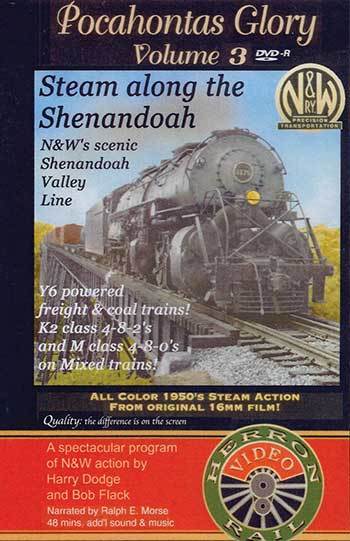This is an image of an advertisement or poster for a DVD titled "Pocahontas Glory, Volume 3." The focal point of the image is a black or gray steam locomotive prominently positioned in the center, traveling over a bridge on the N&W Scenic Shenandoah Valley Line. The train, depicted in vivid colors from original 1950s 16mm film, includes several cars, including a brown boxcar visible in the background. 

At the top of the poster, in black and beige text, it reads "Pocahontas Glory, Volume 3, DVD-R." Beneath this, against a blue backdrop, the text "Steam Along the Shenandoah, N&W Scenic Shenandoah Valley Line" is displayed. Additional information in the lower left corner describes the featured trains: "Y6 Powered Freight and Coal Trains, K2 Class 4-8-2s and M Class 4-8-0s on Mixed Trains." 

The bottom of the poster highlights "All Color 1950s Steam Action from Original 16mm Film" and states, "Quality. The difference is on the screen" in white text against a black background. Against a red background at the very bottom, white text promotes "A Spectacular Program of N&W Action by Harry Dodge and Bob Flack," narrated by Ralph E. Morse, lasting 48 minutes with additional sound and music. On the right side, an emblem resembling a wheel with "Hair and Rail" and "Video" within its spokes adds a distinctive touch to the design.